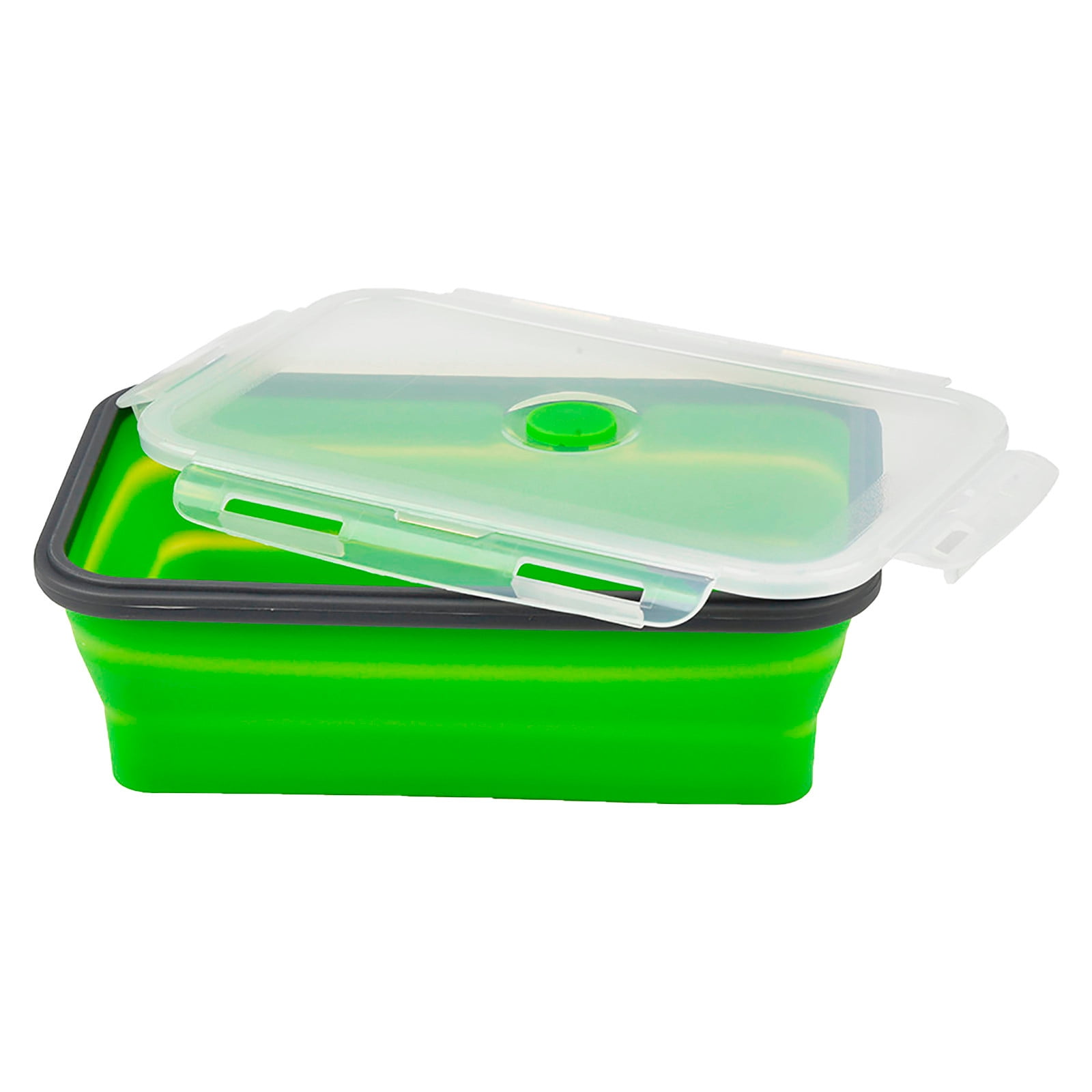This image features a lime green, rectangular, collapsible Tupperware container set against a white background, designed in a style often seen in product advertisements. The container is made of plastic and has a gray trim around the top rim for sealing. It is adorned with two yellow stripes along its sides. 

The translucent, clear lid lies atop the container at an angle, revealing the interior. The lid itself has a green circular button in the center, which matches the container's color. This button likely serves to secure the lid more tightly, maintaining the freshness of the contents inside. There are four tabs or prongs on the lid—one on each side—that snap onto the container to ensure a tight seal. The design suggests that the container can store up to four cups of contents and can be collapsed flat for convenient storage.